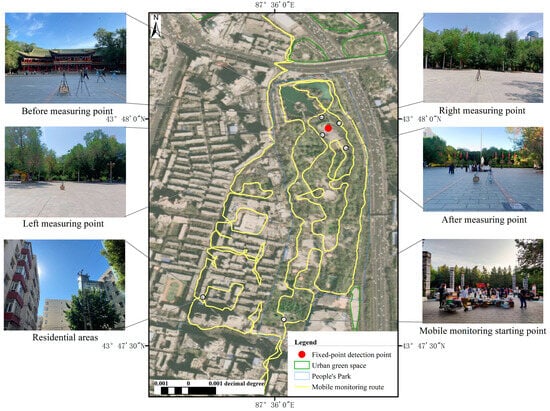This image is a detailed collage consisting of seven photographs. The centerpiece is an aerial photograph of a landscape that appears to be a village or a subdivision. This photograph has various areas outlined in yellow, green, and gray, identifying different features. The yellow outline marks the mobile monitoring route, the green outline indicates urban green space, and the gray outline indicates People's Park. There is a red dot which denotes a fixed point detection point, and a legend in the bottom right corner offers further details, although it is somewhat difficult to read. 

On either side of this main aerial photograph, there are three smaller photographs stacked vertically. 

- On the left side:
  - The first image is captioned "Before Measuring Point."
  - Below it, another image is labeled "Left Measuring Point."
  - The third image is captioned "Residential Areas."

- On the right side:
  - The top image is labeled "Right Measuring Point."
  - The second image is captioned "After Measuring Point."
  - The final image at the bottom is the "Mobile Monitoring Starting Point."

All six side images appear to be outdoor photographs, showcasing various parts of the area, potentially correlating with points along the mobile monitoring route. The photographs are vibrant and in color, depicting various aspects of the landscape and community activities. The central aerial photograph, marked with detailed outlines and labels, serves as the focal point of the composition, providing a comprehensive overview of the measured area.